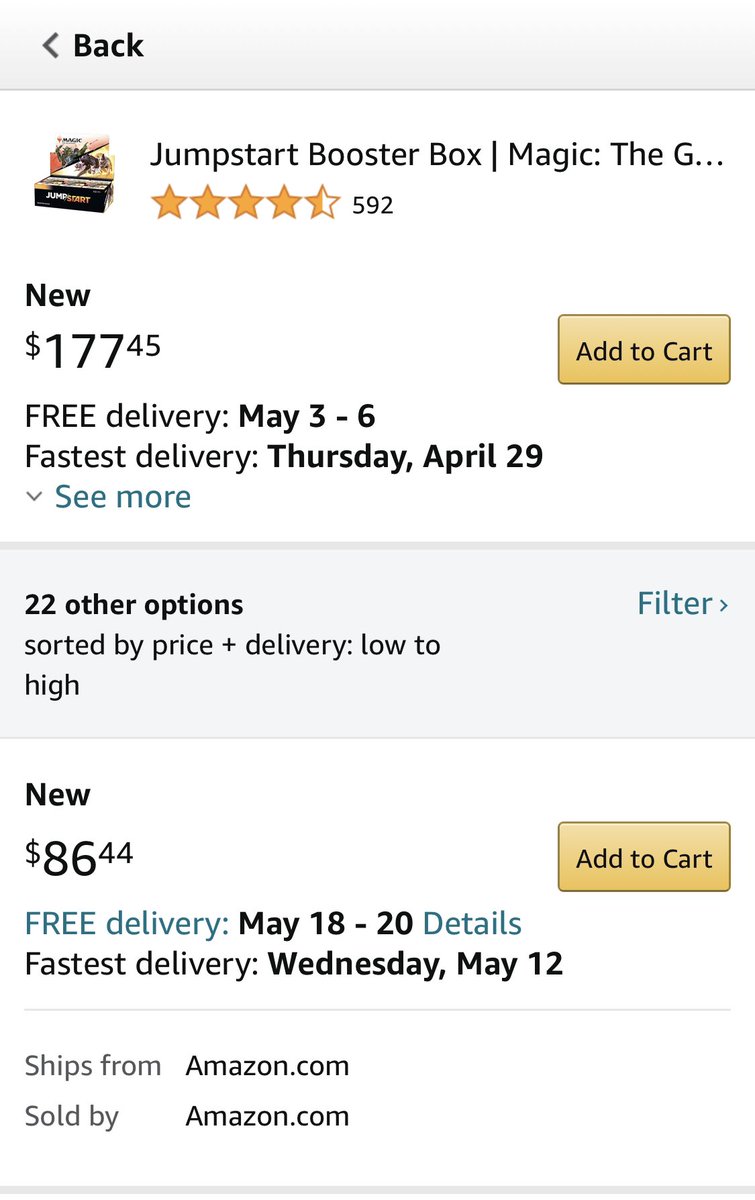The screenshot depicts an Amazon product page as viewed on a mobile device, indicated by the tall rectangular shape of the image. At the very top, there is a gray background with the word "Back" and a left-pointing arrow in black text, which is a common navigation feature.

Below this header, there are two product listings. Separating the two listings is a gray box containing the text, "22 other options sorted by price plus delivery low to high."

The first listing is for a Jumpstart Booster Box from the card game Magic: The Gathering. The product has an average rating of 4.5 stars based on 592 reviews. The image accompanying the listing shows a cardboard box with various graphics related to the game. This item is priced at $177.45 and is marked as new. An "Add to Cart" button is positioned on the right side of the listing. Additional delivery information indicates free delivery between May 3rd and May 6th, with the fastest delivery option being Thursday, April 29th.

The second listing, also described as new, is priced at $86.44. Free delivery for this item is available between May 18th and May 20th, with the fastest delivery option being Wednesday, May 12th.